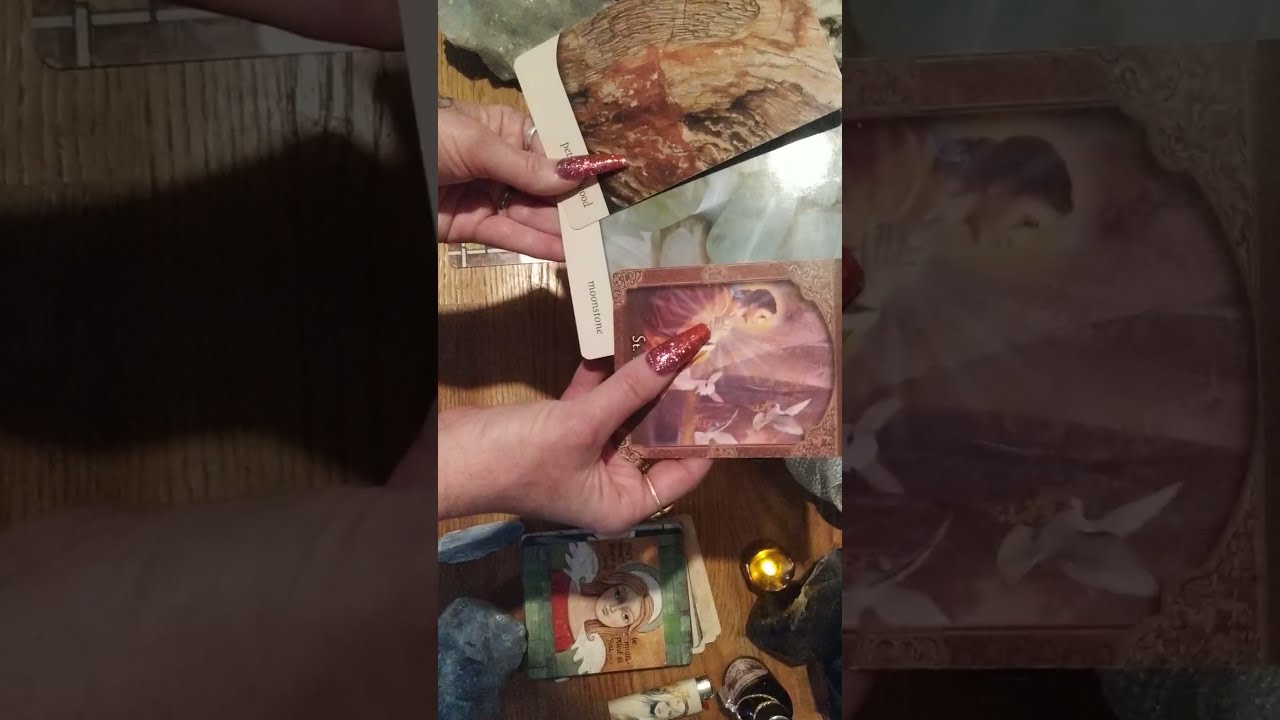The image depicts a close-up of a woman with exceptionally long, red, glittery fingernails holding two tarot cards. The woman's left hand holds a card with a fiery, waterfall-like scene composed of red, orange, and yellow hues against a rocky, brown background. Her right hand holds a card bordered in brown, featuring an angel with dark hair and a red cloak looking up at a white dove, with a white sheep beside the angel. The cards are not easily readable as they are held at an angle and away from the foreground. Additional cards are scattered on a brown wooden table beneath her hands. Among these, a card with an angel with blonde hair, white wings, a red shirt, and green accents is visible. The table also contains a bottle with a white label, a white lighter with a sketched face, a lit yellow candle, and several black and white crystalline rocks. The scene is set indoors, and the image appears to have grayed-out edges, with a vertically centered bright section focusing on the woman's hands and the tarot cards.